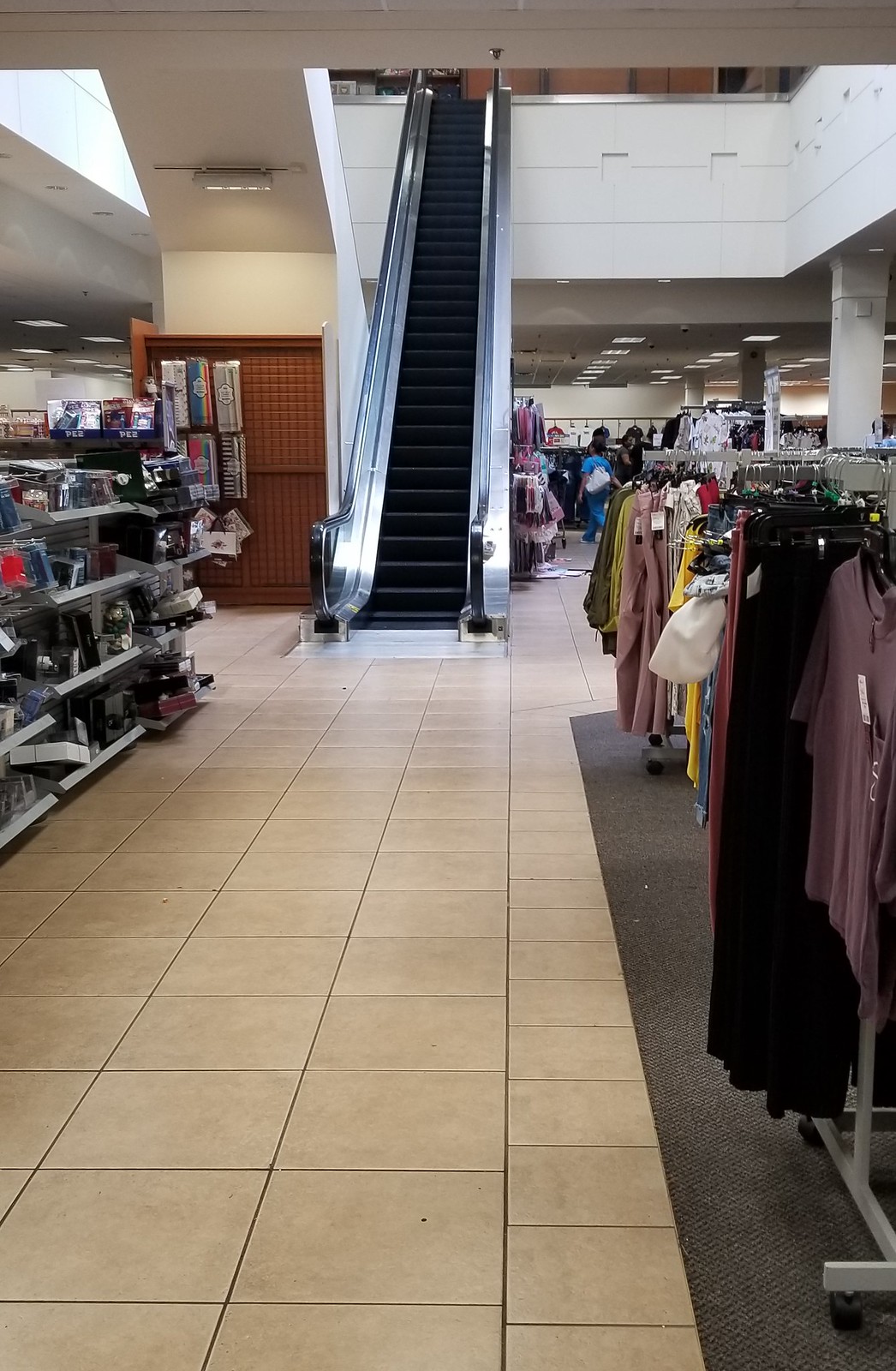This color photograph captures the bustling interior of a modern shopping center. The foreground features a tiled floor with a beige design prominently placed front and center. At the heart of the image, an escalator with black steps and translucent gray rails ascends towards a mezzanine level obscured by a gray ceiling. 

To the left of the escalator, shelves display an array of smaller objects, suggesting a variety of merchandise available. To the right, clothing racks showcase an assortment of apparel. Among the clothing, a distinctive reddish-grey top stands out near the edge of the frame, accompanied by a white bag and garments in yellow and pink hues. These racks are situated on a gray mat, contributing to the organized layout of the store. In the background, a few shoppers meander through the space, their heads just visible, adding a sense of liveliness and activity to the scene.